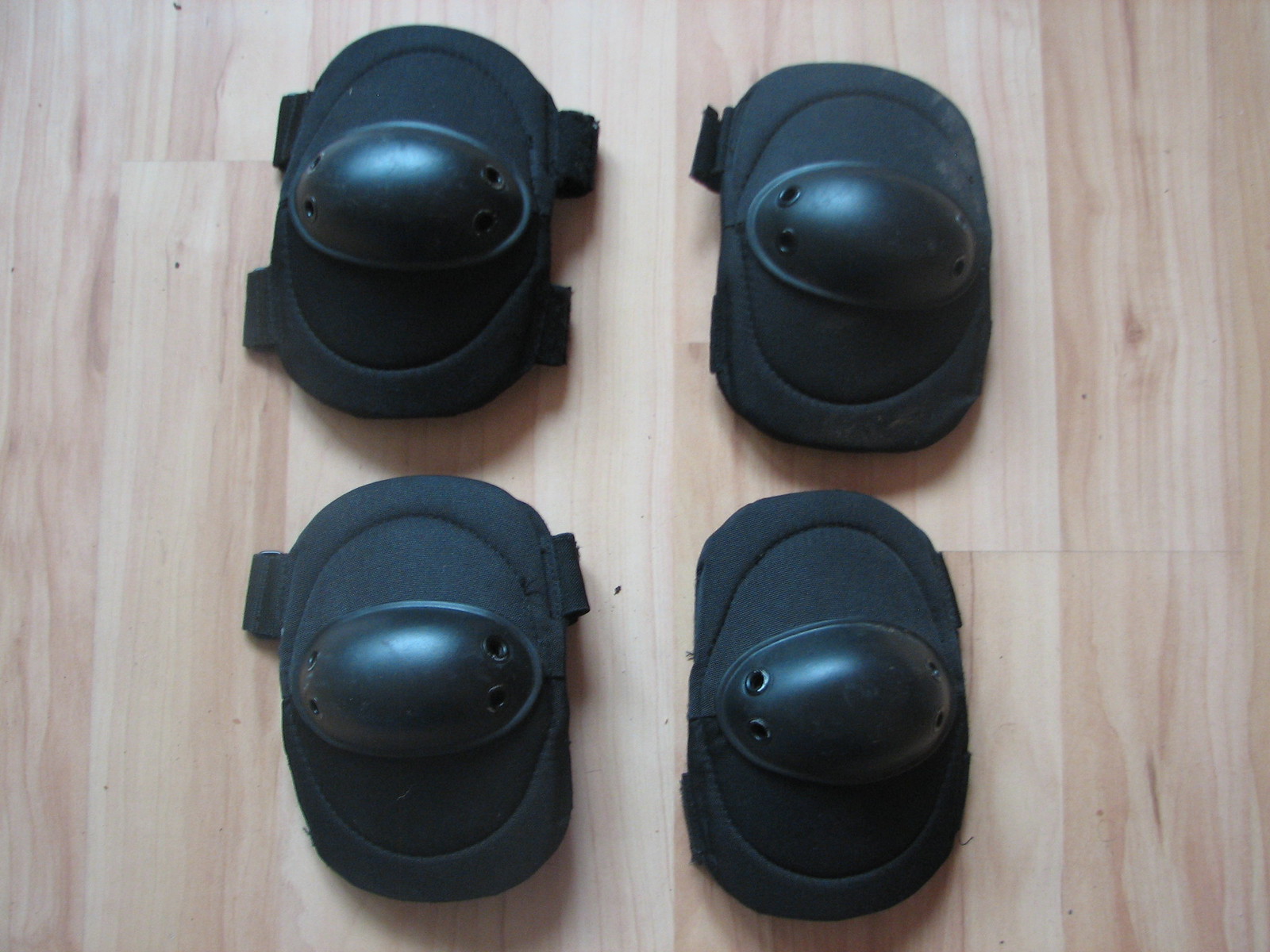The image shows a close-up of two pairs of black knee or elbow guards, likely designed for light, recreational activity such as skateboarding rather than heavy-duty work. Each guard consists of a soft black fabric backing equipped with Velcro straps at both the top and bottom for secure fastening. In the center of each pad, there is a hard, oval-shaped protective plate with a wide cup and two side recesses. The guards are arranged on a light-colored hardwood or laminate floor, giving a clear view of their construction and materials. This setting emphasizes the basic protective function of these pads, perhaps intended more for the peace of mind of parents than for rigorous use.